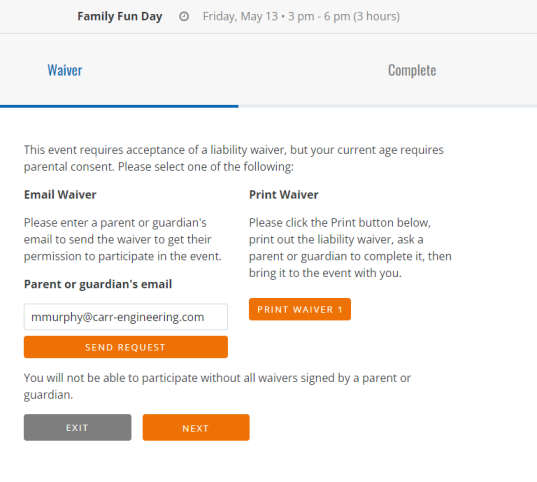The screenshot depicts a waiver page for an event titled "Family Fun Day" scheduled for Friday, May 13, from 3 p.m. to 6 p.m. (a total duration of three hours). The page informs that participation in the event requires acceptance of a liability waiver, and since the current user's age necessitates parental consent, they must choose one of the following options:

1. **Email Waiver**: The user is prompted to enter a parent or guardian's email address in the provided box to send the waiver form for permission to participate in the event.
2. **Print Waiver**: The user can click the "Print Waiver" button to print out the form, which must then be completed by a parent or guardian and brought to the event.

A warning below these options emphasizes that participation is only possible if all waivers are signed by a parent or guardian.

The webpage has a color scheme featuring white, off-white, bright blue, dark gray, and light gray tones. The main text appears in light gray, while headers are in dark gray. The word "waiver" at the top is displayed in bright blue. Interactive elements such as the "Print Waiver" and "Send Request" buttons are orange with white text. At the bottom of the page, there is a gray "Exit" button and an orange "Next" button with white text.